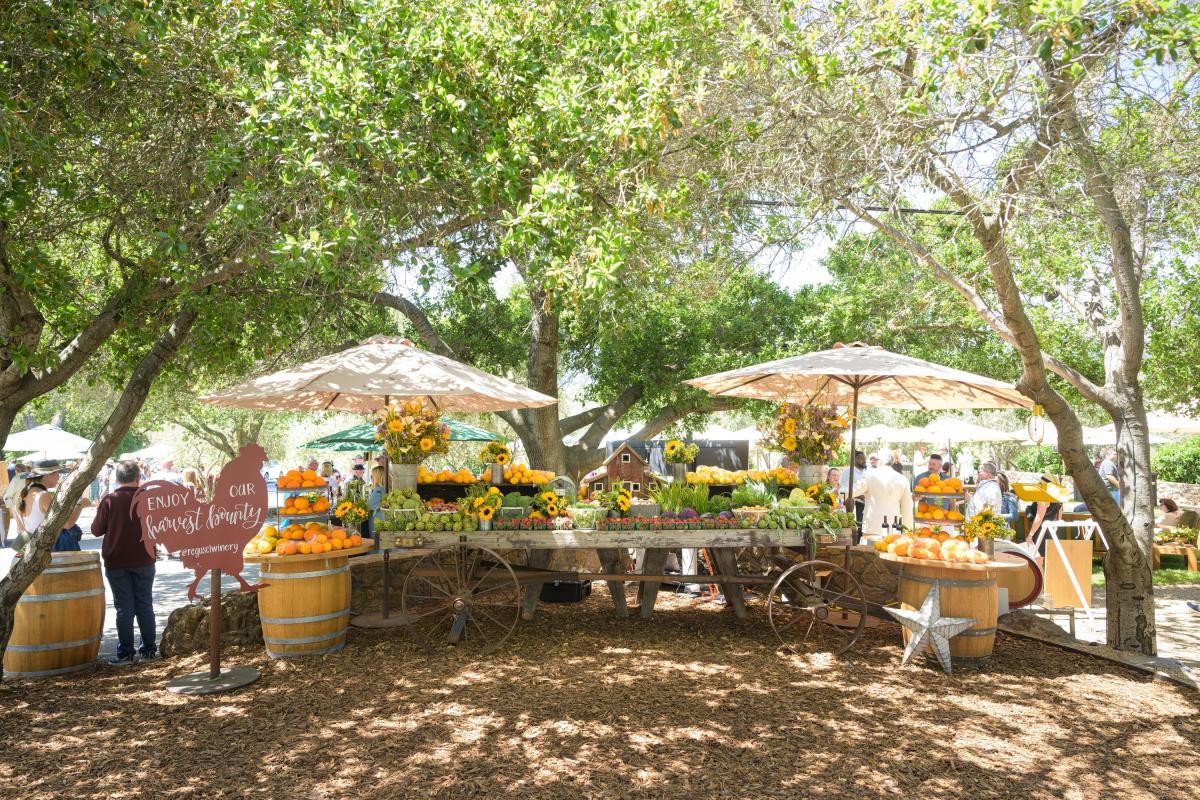This image captures a wide-angle shot of a vibrant booth at an outdoor farmer's market, set on a ground covered in leaves. The central feature is a long, rustic table crafted from an old wooden wagon, complete with large, spoked metal wheels on either side. The table surface is adorned with an abundant display of sunflowers, arranged in tall vases, pots, and scattered loosely across the table. 

At both ends of the wagon, two white parasol umbrellas provide shade, flanked by light wood barrels banded with silver metal. The barrel on the right has a silver star leaning against it and contains an array of oranges, while the left barrel holds layers of oranges, lemons, and possibly tomatoes and onions. 

Adding to the festive atmosphere, a cutout sign in the shape of a chicken on the right side bears the message "Enjoy our harvest, family." Behind the wagon, people mill about, and several other tables with umbrellas offer various fruits, vegetables, and flowers. Trees line the scene to the left and right, their shade partially covering the wagon and enhancing the rustic charm of this bustling market.